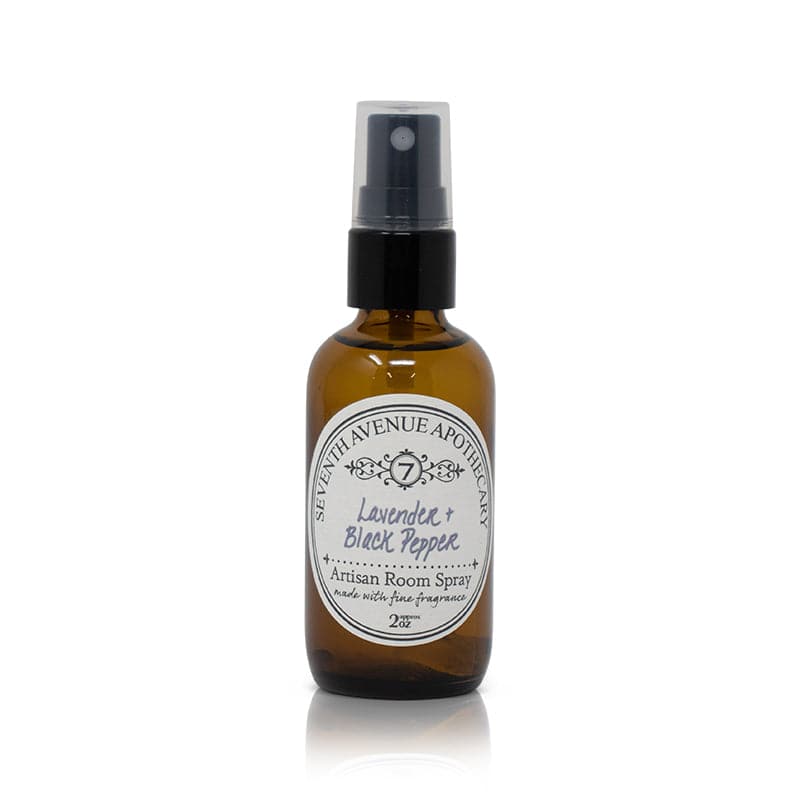This photograph depicts a small, clear bottle with a brown tint, possibly made of glass or plastic. The bottle has a black plastic spray pump, covered by a clear cap, revealing a straightforward spray nozzle mechanism. The liquid inside is visible due to the bottle's translucency. The bottle features an oval, adhesive label marked with intricate details. At the top of the label, it reads "7th Avenue Apothecary," with the number "7" encircled and adorned with ornate lines, all printed in a script-like or silver-colored font. Below this, the scent "Lavender + Black Pepper" is prominently displayed in a lavender hue, followed by a dotted line. The label further identifies the product as an "artisan room spray made with fine fragrances," concluding with a notation of "2 OZ for houses" in smaller text.